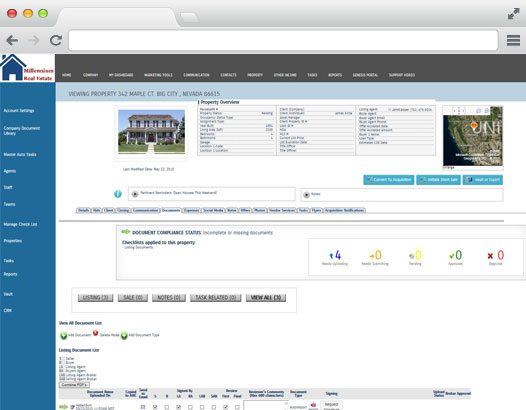This screenshot captures a website interface, detailing both its browser and webpage elements. At the top of the browser window, a gray bar features three small, colorful circles in the upper left corner—red, green, and yellow—reminiscent of typical window control buttons. On the upper right, black arrows are visible. Beneath the gray bar is a blank address bar, suggesting the absence of a URL. Adjacent to the address bar, on the right, are three gray horizontal lines, likely representing a menu icon. To the left of the address bar, navigational buttons are positioned in sequence: a back button, a forward button, and a refresh button.

The main content of the webpage is undersized, rendering the text unreadable. However, the left-hand side features a vertical blue rectangle with white text aligned vertically. On the right, the webpage displays a predominantly white screen with images of various houses and small graphs. Among these images, a picture of a house and an outline of California can be discerned, surrounded by substantial text that remains too small to interpret. The overall screenshot is notably small, limiting the clarity of the depicted elements.